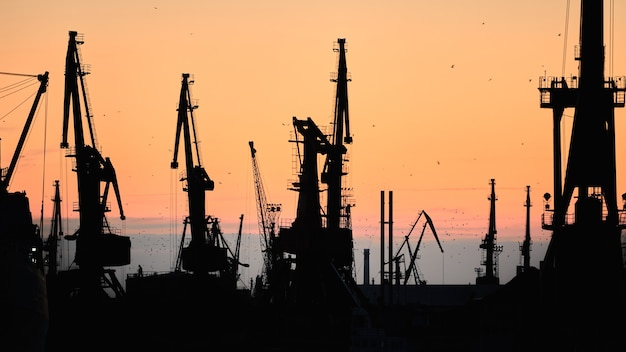The image captures a dusk scene of an expansive, flat oil field silhouetted in darkness. A line of oil drilling machines, resembling cranes with their tall, thin structures and hinged, downward-hanging metal arms, are prominently featured in the photograph. These oil rigs, both in the foreground and stretching into the distance, appear as black silhouettes against a vibrantly colored sky. The background transitions from a deep orange and pink near the horizon to a darker blue closer to the land. Filament-like power lines are visible to the right, cutting through the serene, yet industrial landscape. The lighting obscures specific details of the machinery, casting them into shadow and emphasizing their stark, imposing presence against the striking, photorealistic backdrop.